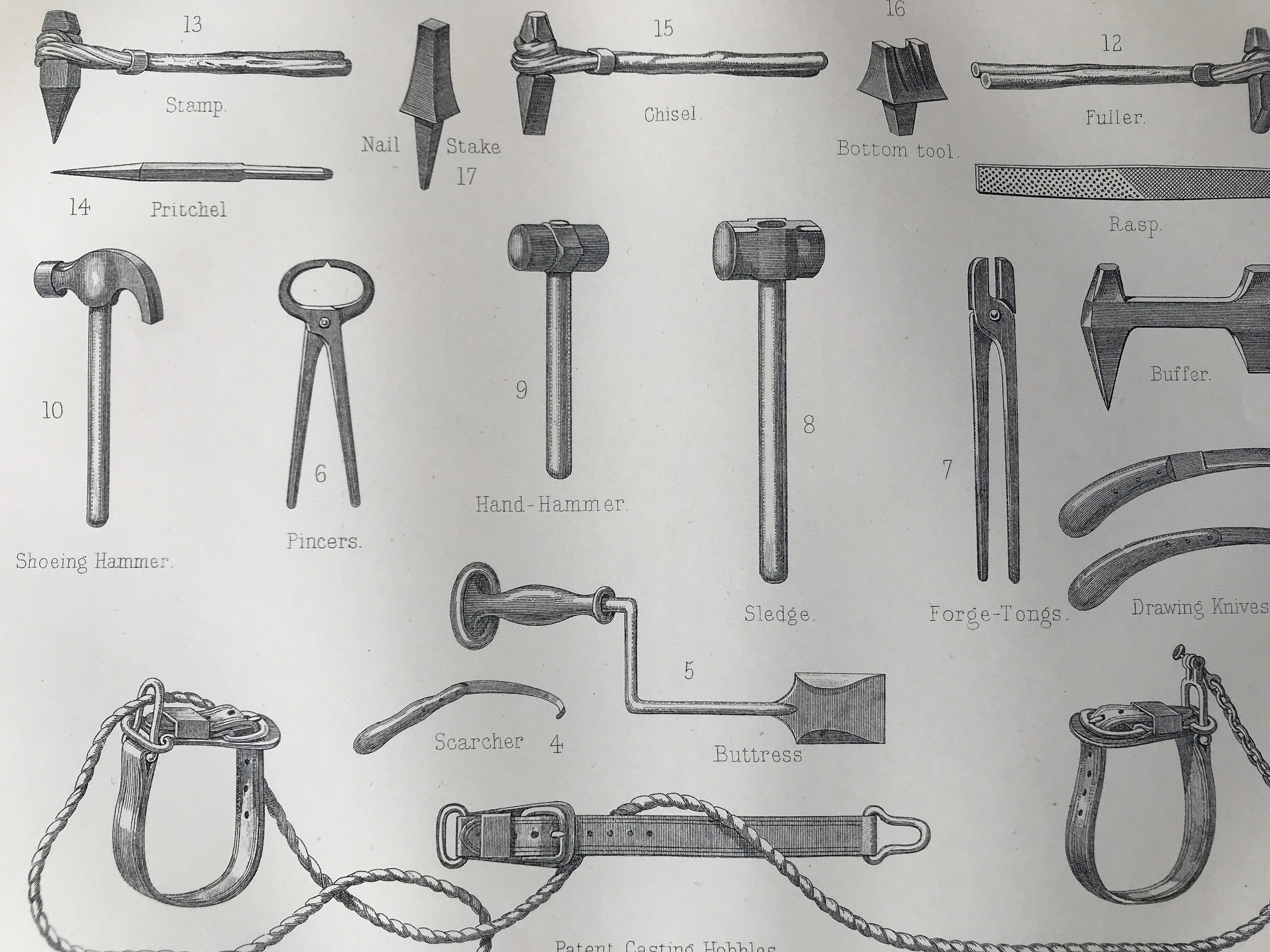This black and white image is a detailed, rectangular sketch of various metal tools, drawn in pencil or light ink against a gradient background that shifts from off-white on the left to a grayer tone on the right. The tools are meticulously laid out in rows from top to bottom, each accompanied by numeric labels and brief descriptions. It features items such as a stamp (13), a pretzel (14), a shoeing hammer (10), pincers (6), a hand hammer (9), a nail stake (17), a chisel (15), a bottom tool (16), a fuller (12), a rasp buffer, drawing knives, forge tongs (7), a sledge (8), a scratcher (4), a buttress (5), and other related equipment. The bottom of the image has a complex arrangement of a strap with foot straps on either side and a winding rope, culminating in a chain on the right. A partially cut-off phrase, "patent casting hobbies," appears at the bottom, suggesting either a tagline or a company name, although only the top half of the words is visible.